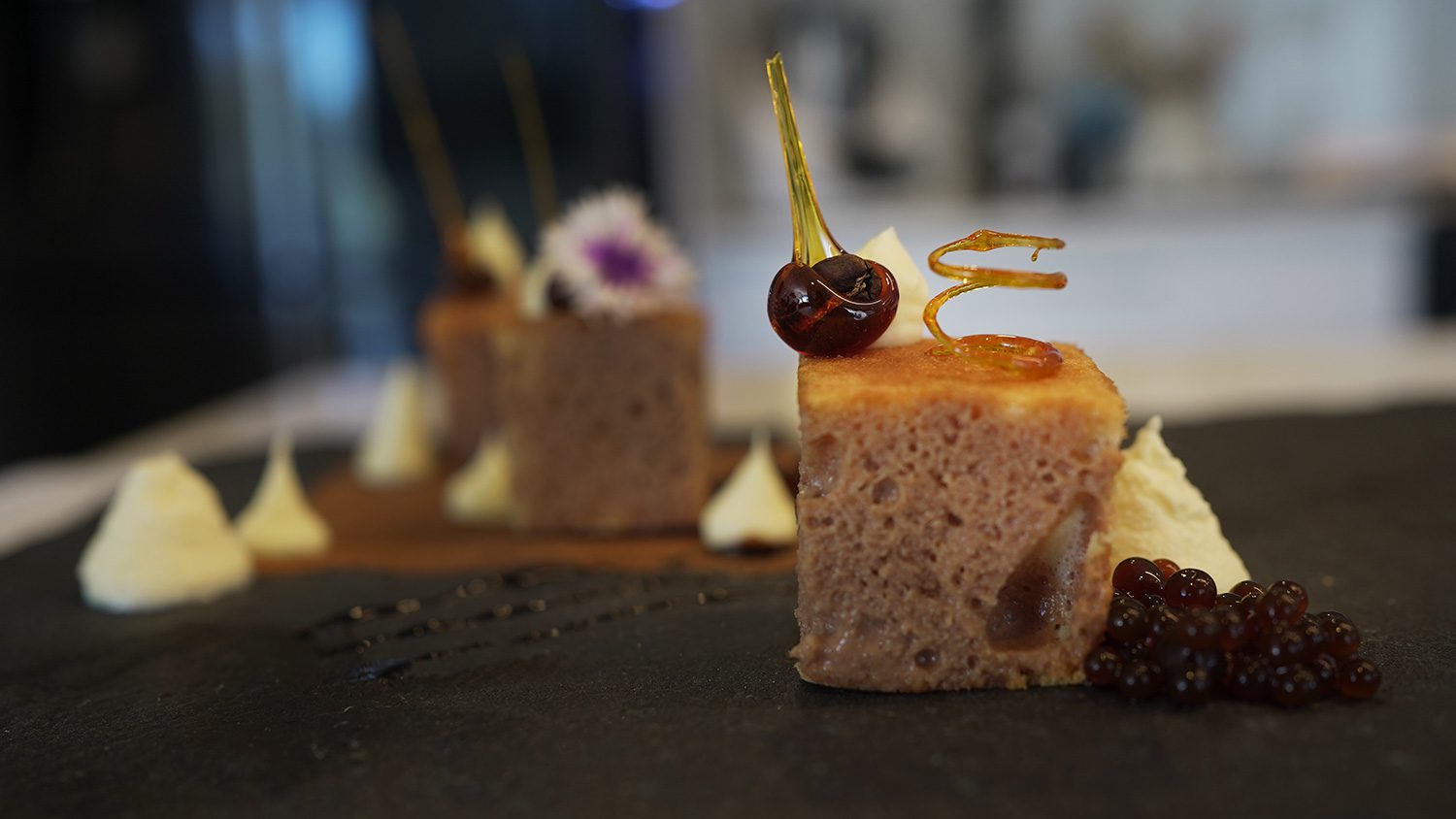The image showcases a professionally captured, intricately plated dessert. Dominating the black platter in the spotlight is a porous, light brown cake cube adorned with a glossy, candied cherry, complete with a vibrant green stem and succulent red fruit. Crowning the cake is a crisp, spiraled decoration that appears to be caramelized honey. To the bottom right of the cake rests a dollop of white cream, potentially whipped cream, accompanied by small, dark purple spheres resembling miniature grapes or mochi. The background, intentionally blurred, reveals two additional cake pieces; one decorated with a pink and white flower and another indistinguishable due to the blur. Scattered across the scene are multiple delicate, triangular peaks of whipped cream. The overall composition is a harmonious blend of black, white, gray, brown, yellow, red, green, purple, and off-white tones, forming a visually captivating dessert display without any text.